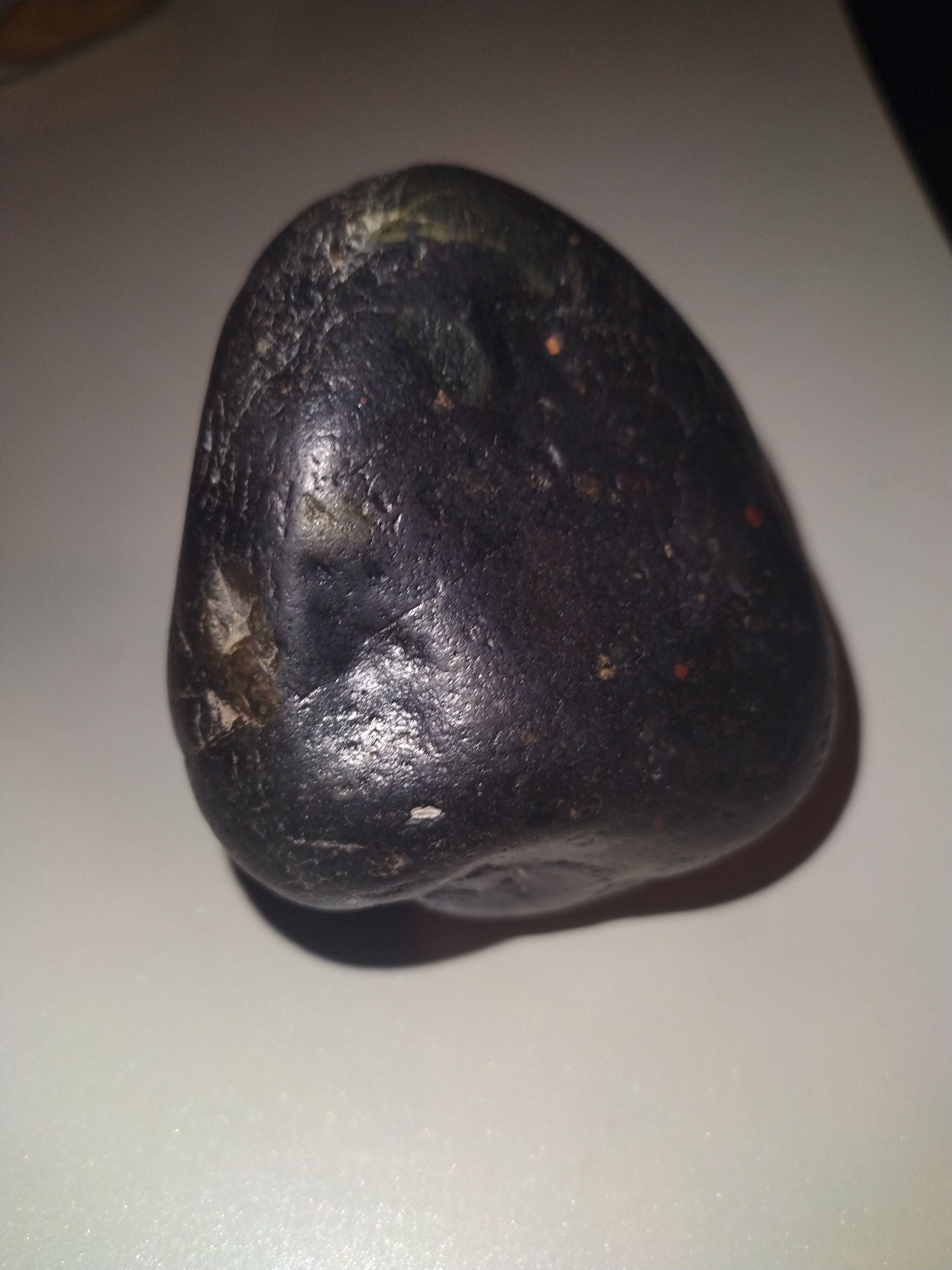In this detailed indoor photograph, a single large, smooth, black rock—potentially obsidian or a polished volcanic rock—sits prominently at the center of a white tabletop or countertop. The rock, about the size of an egg or slightly larger, showcases a mix of colors including blacks, grays, browns, reds, oranges, greens, and beige. Its mostly polished surface suggests natural water erosion, likely from rivers or beaches, rather than machine-polishing. The rock is triangular with rounded edges, presenting a pointed tip facing north. It features creases, lumps, and a shiny lower left side highlighted by the flash. Shadows beneath the rock and light tan indentations toward the top and left side, accompanied by red dots on the right, add texture and depth to its appearance. The background is a light gray to nearly white, with blacked-out edges in the upper left and right corners, giving a clear and focused documentation of the rock.